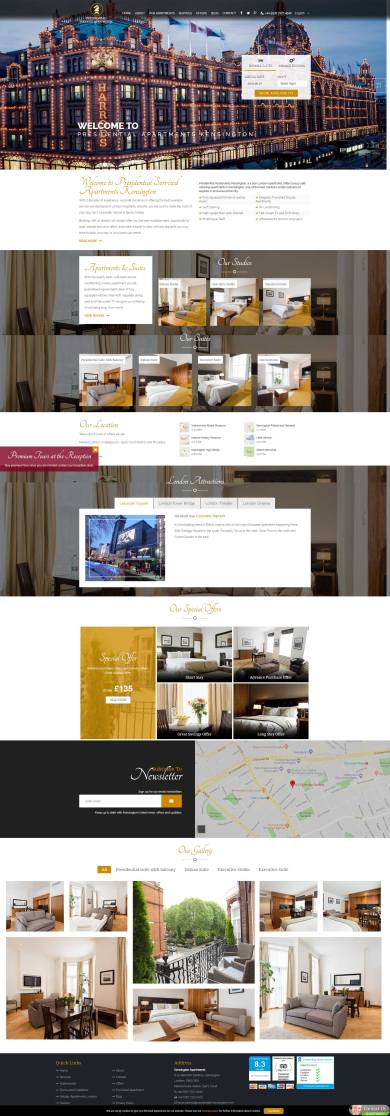A scrolling screenshot of an extensive web page, capturing eight distinct sections, a navigation bar at the top, and a comprehensive footer. The hero image at the top showcases Buckingham Palace with the welcoming message "Welcome to" prominently displayed, followed by additional white text. The third section appears to feature various beds, possibly indicating room options or accommodations. The fourth block contains images that are difficult to discern but seem related to room interiors. Similarly, the fifth block includes more images of beds. The sixth section highlights a map for navigation purposes. The seventh block showcases different pieces of furniture that may be available in the rooms. Finally, the footer spans three columns, listing various links and supported credit card payment options. The navigation bar at the top of the web page is black with white text for the menu items.